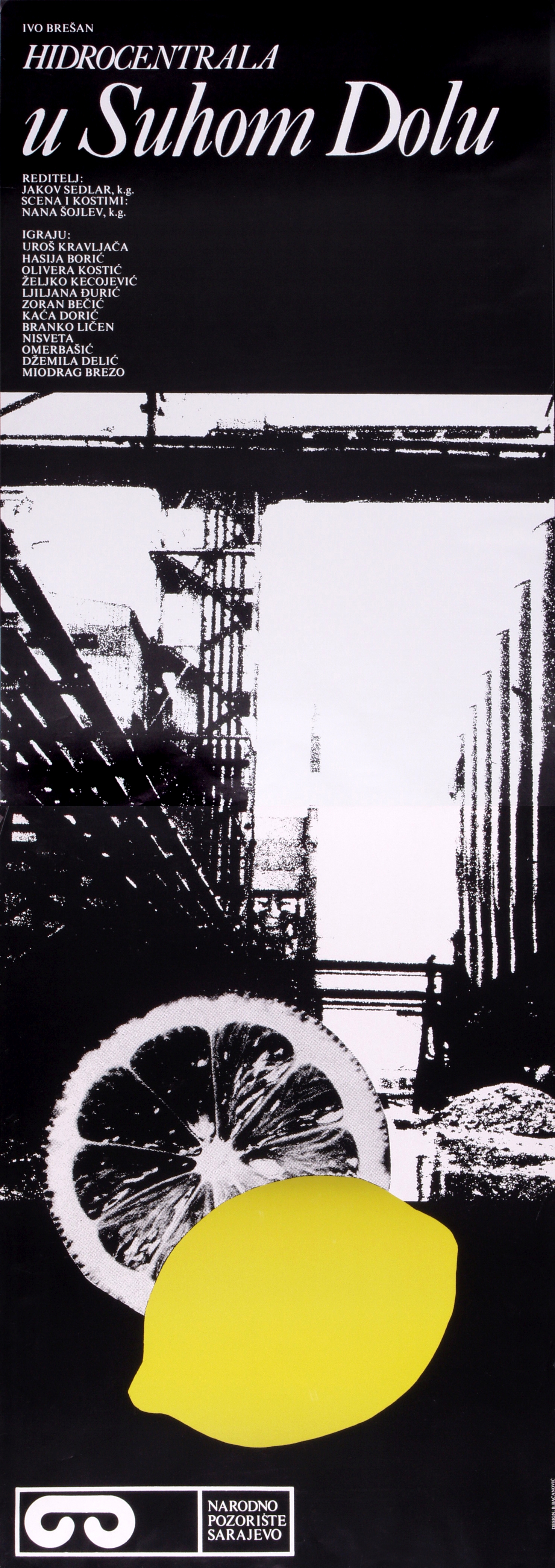This poster is a modern abstract graphic art piece featuring a narrow vertical rectangular format with a solid black background, especially prominent at the top and bottom. At the top, a block of black houses white text in a foreign language, reading "Hydrocentrala" followed by "U Suhamdolu" in larger letters, with a list of names or credits below in smaller white, left-aligned print. Dominating the center is a black-and-white image, likely a photograph, depicting a cityscape with a high-rise work platform, bridge, or industrial area under a sky. This central image exudes an urban, industrial atmosphere. At the bottom, a bold, yellow solid lemon stands out vividly against the monochromatic backdrop, partially obscuring a black-and-white cross-section of a lemon behind it. A small white icon resembling an eye with additional text, "Narodino Pozariste Sarajevo," appears in the bottom left corner. This mixed-media poster seamlessly blends photograph and digital drawing, with the yellow lemon adding a striking focal point amid the grayscale scene.